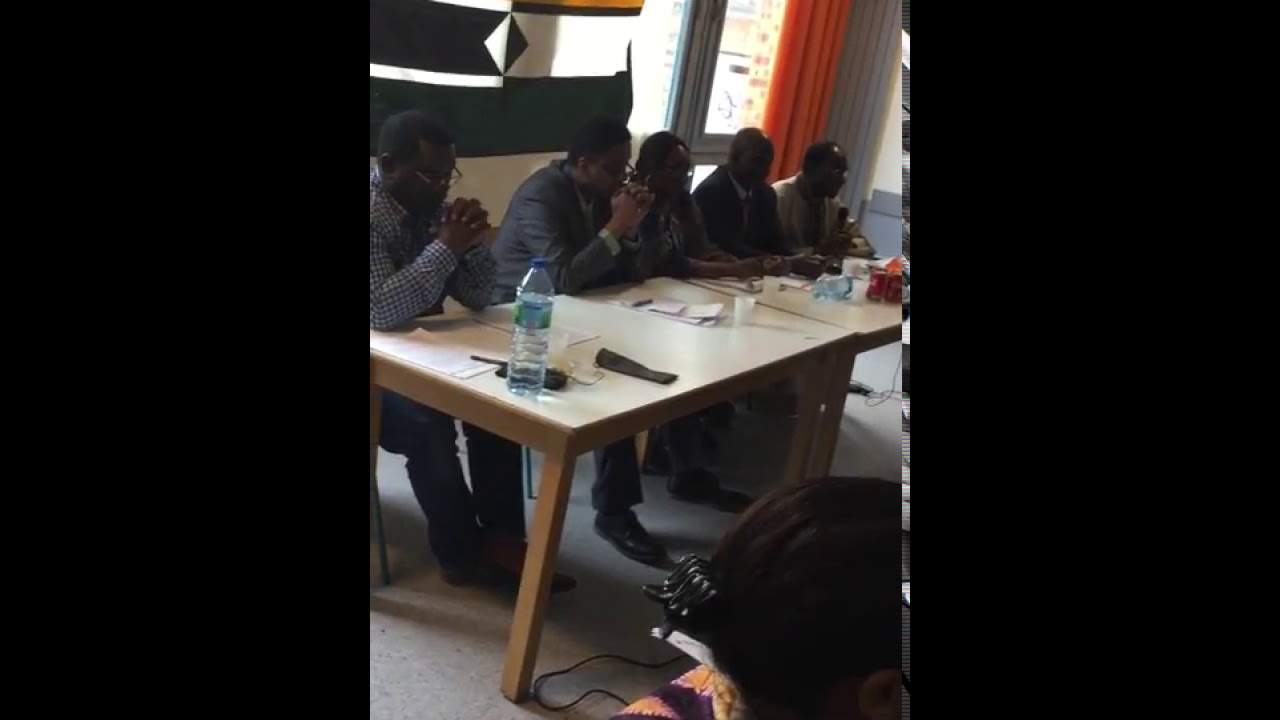In the center of this indoor image, five people of African descent sit behind a light tan table, which appears to be two tables pushed together. The group consists of four men and one woman, who is positioned in the middle. Three of the men have their hands clasped, appearing to be in prayer. On the table, there are scattered papers, a tall bottle of water located on the left side, and a possible telephone or walkie-talkie. The man furthest to the right might be holding a microphone, though their features are not clearly visible due to shadows. Behind this man, there is an orange curtain on the left side and a light gray curtain on the right. In the bottom right corner, the back of a woman's head is visible; she has dark brown hair secured with a black banana clip, along with glimpses of purple and orange fabric from her shirt. The setting suggests a meeting or discussion, with a window and potential black-and-white banner partially visible in the background.